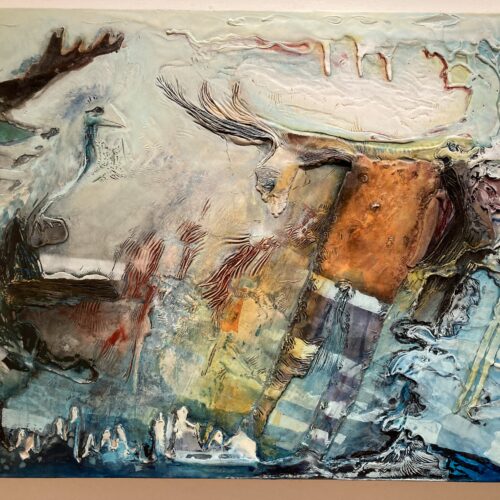The image is a detailed, textured painting created on a flat canvas-like material, featuring a heavy application of paint that gives a distinct 3D effect. At the top, the canvas is bordered by white, while the bottom edge sports a brown border. The focal point on the right side is a stylized depiction of a moose with large antlers, viewed from its midsection to its head, looking to the left. A stylized blue bush is painted in front of this moose, and above it, the sky is rendered in white with various drips coming down, enhancing the abstract atmosphere of the piece. 

On the left side, there is a smaller, hornless moose gazing back at the larger antlered moose. Perched on top of this hornless moose, there is a bird-like shape painted in white, adding a layer of intrigue. Additionally, there are elements which could be interpreted as ocean or river scenes with boats and people, as well as splashing waves transitioning into a creature, hinting at a sense of motion and life. 

The overall style is abstract and somewhat surreal, blurring the lines between natural elements and imaginative forms, possibly even merging human forms with those of animals. The mix of dense paint layers and artistic techniques creates a rich texture, providing depth and a multifaceted viewing experience.